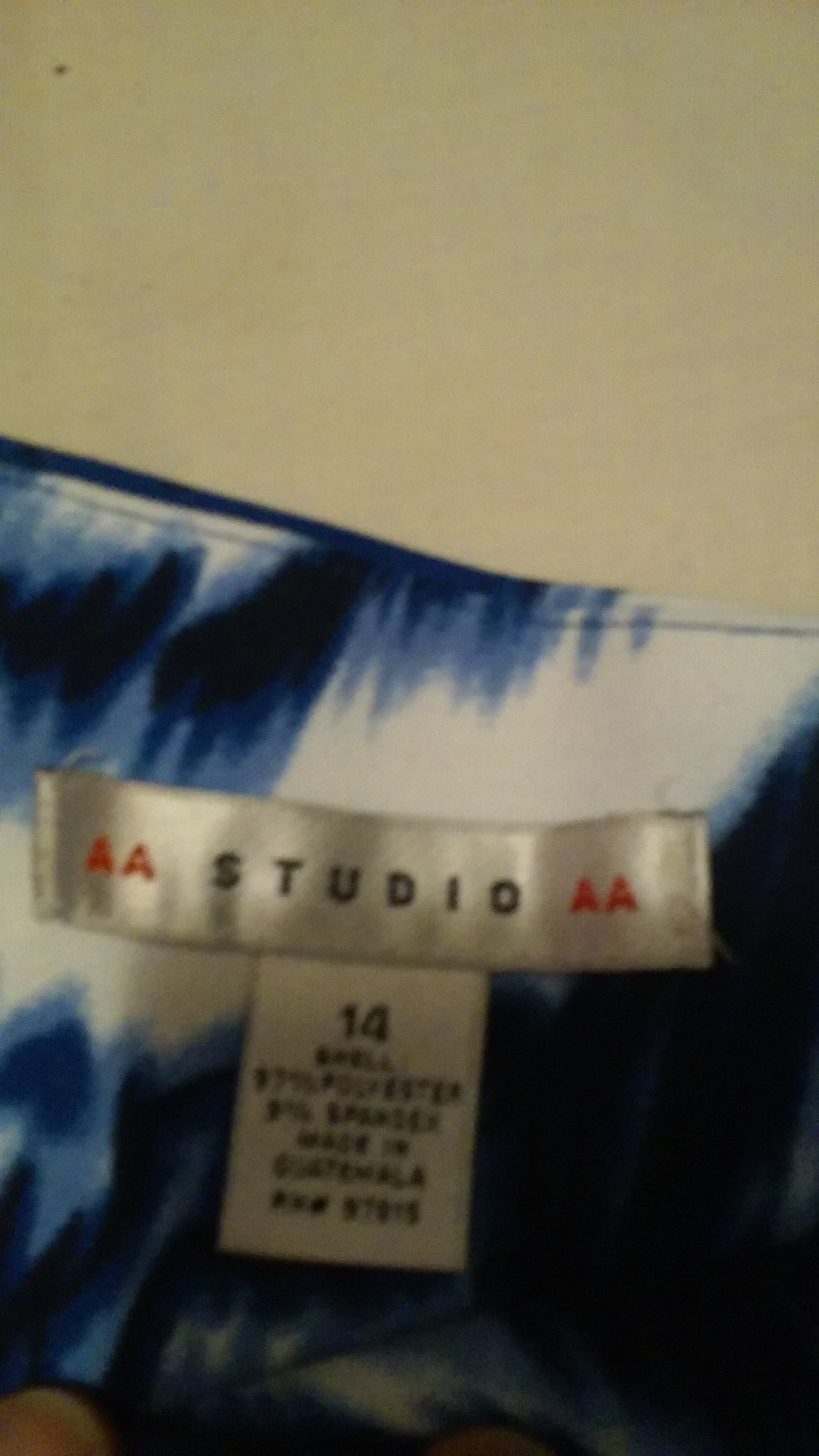The image showcases a piece of clothing with a distinctive tie-dye pattern in shades of dark blue, light blue, and white, featuring zigzag lines, shading, and stripes. The focal point is a white rectangular label that prominently displays "AA Studio AA" with "AA" in red and "Studio" in black. Attached to this label is a smaller square tab indicating a size 14, along with information that the garment is composed of 97% polyester and 3% spandex, manufactured in Guatemala. The clarity of the text on the label is somewhat compromised, making it difficult to read all the details clearly. Above the fabric, the background transitions to a light gray wall. This appears to be an article of women's clothing, potentially a skirt or dress based on the visible fabric design.